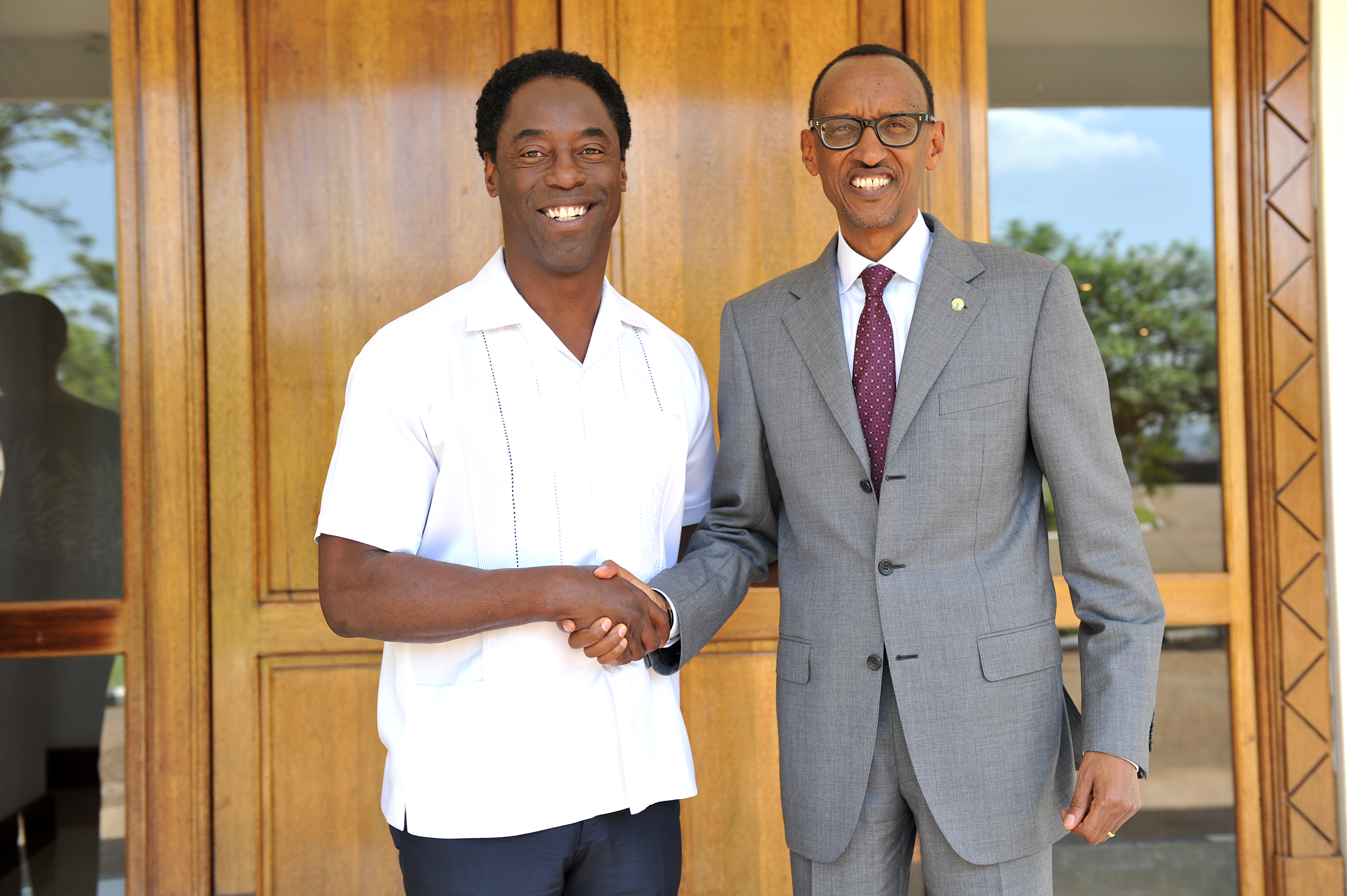In the photograph, two distinguished African descent gentlemen are shaking hands in front of a wooden door with glass panes. The man on the left, who appears middle-aged with short black hair, is wearing a white short-sleeve, button-down shirt, and dark blue pants. The man on the right, who seems older, is dressed in a gray suit with a purple tie featuring white dots and black spectacles. Both men are smiling, their mouths slightly open, exuding a professional and approachable demeanor. The background contains glass windows on either side of the door, reflecting a serene blue sky, trees, and a hint of the ground. Additionally, the reflection of another person is visible on the left side of the glass.